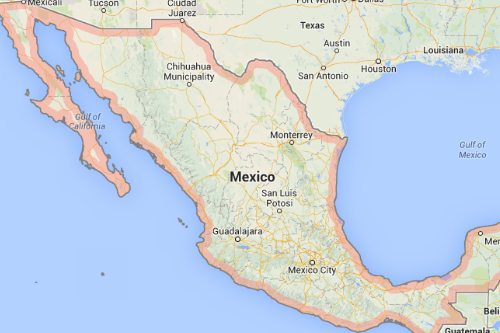A cropped, low-resolution image of the country of Mexico extracted from a broader world map. The map exhibits noticeable artifacting around some of the text. In the upper portion, U.S. cities like Austin, San Antonio, and Houston in Texas are visible. The Mexico border is distinctly highlighted in a pinkish-red color. Across Mexico, major cities are marked, including Chihuahua Municipality, Monterrey, San Luis Potosí, Guadalajara, and Mexico City. To the right of these, the Gulf of Mexico is clearly labeled, and to the left, the Gulf of California is also marked. Bordering states from the U.S., such as Arizona with Tucson, are annotated at the northern edge. Prominent border cities within Mexico, such as Ciudad Juárez, are noted. The land is color-coded in shades of yellow to green, with various roadways and waterways intricately mapped. The water regions, specifically the Gulf of California and the Gulf of Mexico, are depicted in a light pale blue hue.